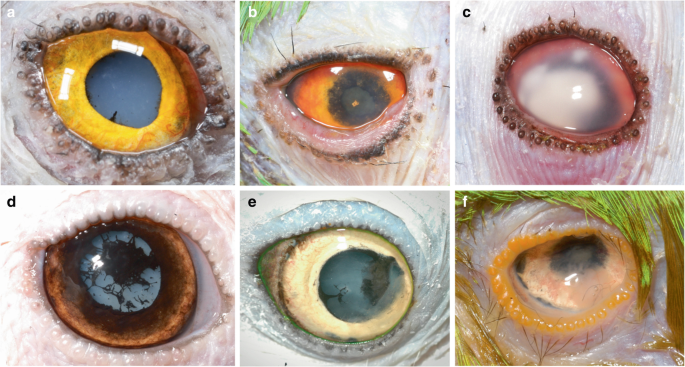This image displays a collection of six close-up photographs of various animal eyes, arranged in two rows of three. Each photograph is labeled in the top left corner with a letter, from A to F. 

- **A**: This eye has a vibrant yellow iris with a black pupil, suggesting a bird species.
- **B**: Featuring an orange iris with a black pupil, this eye might also belong to a bird.
- **C**: The eye appears milky white and cloudy, possibly indicating impaired vision.
- **D**: This eye is brown with a large black pupil that nearly fills the eye.
- **E**: It showcases a light yellow iris with a black pupil in the center.
- **F**: This eye has a light orange iris with a black pupil, surrounded by a distinctly orange eyelid and a grassy background.

The eyes are not human, adding an element of intrigue as they might belong to various animals, likely birds given the descriptions.